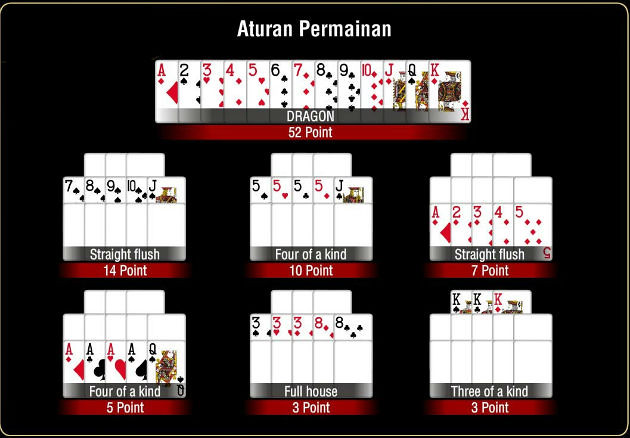This detailed image presents a sophisticated digital graphic of various playing cards meticulously arranged against a stark black background. At the top, the title "Auturin Permian" is prominently written in bold white text, providing a striking contrast to its backdrop. Below this title, an extensive assortment of playing cards is systematically organized in sequential order, ranging from Ace, Two, Three, Four, all the way through to Jack, Queen, and King, effectively representing a full deck.

Beneath this primary layout, a notable black box features the word "Dragon," accompanied by a declaration that it is worth 52 points, signifying a potentially high-value element in the depicted game. Directly below this highlight, there are six additional scorecards, each representing different scoring combinations and values essential to the game's strategy.

From left to right, top to bottom, these scorecards are labeled and valued as follows: "Straight Flush" worth 14 points, "Four of a Kind" worth 10 points, another "Straight Flush" worth 7 points, a second "Four of a Kind" worth 5 points, "Full House" worth 3 points, and "Three of a Kind" also worth 3 points. Each scorecard hosts a unique pattern and combination of playing cards, indicating the multiple ways to score points and the strategic complexity of the game being illustrated. The meticulous arrangement and diverse scoring options suggest a well-thought-out gaming system that emphasizes both order and the significance of different card combinations.